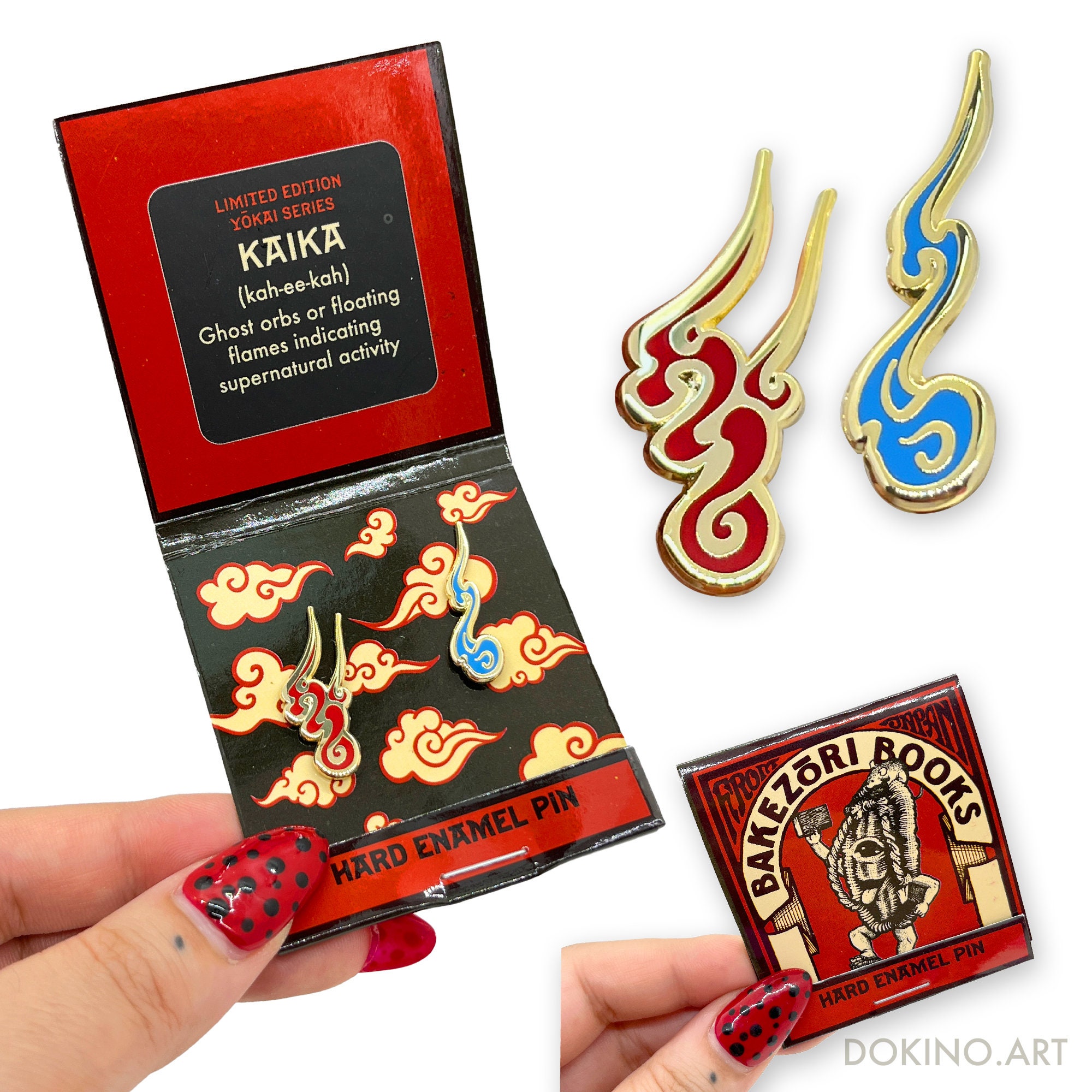The image is a product showcase likely from an online store, presenting limited edition Yokai Series Kaika hard enamel pins. The primary focus is a matchbook-shaped package, prominently held by a hand with red nail polish adorned with black polka dots and a small black dot tattoo on the thumb.

On the left side of the image, the hand is holding the open package. The top half of the package is red with a black label reading "Limited Edition Yokai Series Kaika" along with the description "Ghost orbs or floating flames indicating supernatural activity." The bottom half reveals two enamel pins attached to a black background featuring stylized cream clouds with red borders. These pins are fastened securely, and below them, the text "Hard Enamel Pin" is displayed.

On the top right side of the image, there are enlarged views of the two enamel pins. The pin on the left is red with gold borders, designed as a detailed swirl with intricate gold details, while the pin on the right is blue, also with gold borders, and is more elongated with small gold accentuations.

At the bottom right, the package is shown closed. The red cover features a cream arch labeled "Bakazori Books," with an illustrated happy creature sticking out its tongue and holding a book. This creature, along with a small mouse perched atop, is rendered in a sketch-like style. The bottom text of this closed package repeats "Hard Enamel Pin." Additionally, a faint watermark reading "dokino.art" is visible on the bottom.